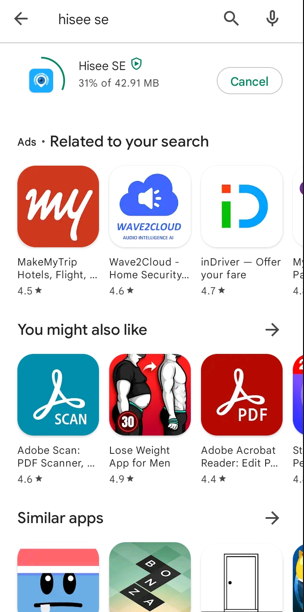This is a detailed screenshot from a smartphone or tablet, displaying a variety of visual elements and interface features. 

At the top in the white bar, there is a black arrow pointing to the right. The central text reads "Hi C, S C, H I S, E E, S E," followed by a black magnifying glass icon and a microphone icon on the right side. Below this is a dark gray line.

To the left, there is a light blue square with a dark blue circle surrounded by white bands. Next to it, a green quarter circle appears with the text "Hi C, S C" in black with capitalized "S C" adjacent to it. There's a green shield symbol with a green triangle inside. Underneath these, it says "31% of 42.91 MB." 

A white button with a gray border is next, containing the word "Cancel" in green. Below this, there's an advertisement section with the text "Related to your search" in black. 

Highlighted within a red square is the word "my" in white cursive, followed by the black text "Make My Trip Hotels, Flights," with three ellipses. Underneath, it indicates a rating of "4.5" with a black star next to it.

Further down, there's a white square with a dark blue cloud icon featuring an audio symbol at its center. Underneath this, it says "Wave to Cloud" and "Wave to Cloud Home Security," rated at "4.6" with a star next to it.

Next is a white square topped with a red square and a longer green rectangle followed by a dark blue half-circle. Below, it says "inDriver - Offer Your Fare," rated "4.7" with a black star. 

The text "You might also like" leads to a dark blue square featuring the Adobe symbol and the text "Scan" below "Adobe Scan PDF Scanner," rated "4.6" with a star.

Following this, there is an image within a red rectangle featuring two versions of a man. One is heavyset with a short-sleeved black shirt, partially showing his stomach, painted white with a beard, wearing black pants with a green band. Next to him is his buffer, shirtless rendition, still adorned in white pants with a green band. A red circle shows "30" in white with a white arrow pointing from the heavier to the buff version.

Finally, the app section for Adobe is shown, featuring the red Adobe symbol and mentions of "PDF" and "Adobe Acrobat Reader," with a rating of "4.4" next to a star. The lower portion displays the edge of another red app with white text, transitioning into purple and blue colors.

At the bottom, under "Similar apps," there is a pink square with white and cyan blue accents featuring black eyes with white dots and a black line. A teal and yellow square with an overturned section reads "BONCA" in white text. On the right, there is a door icon in white with black accents next to a black arrow.